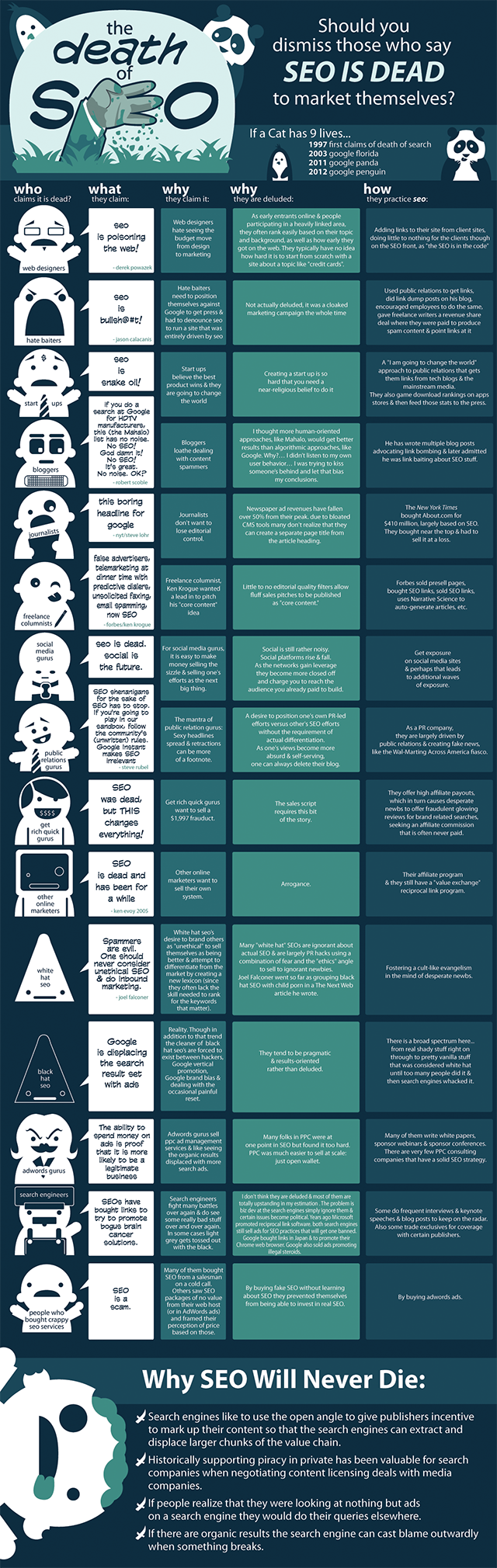In this image, the background is a dark blue, creating a stark contrast with the various elements and text present. Dominating the upper right corner is a piece of white text that reads: "Should you dismiss those who say SEO is dead to market themselves if a cat has nine lives?". Accompanying this text is an image of a cat, reinforcing the metaphor.

On the top left, there's a black and white panda drawing, which adds a whimsical touch. Below this, there's a light green tombstone illustration with the words "The Death of CEO" inscribed on it. Interestingly, the letter "A" in "CEO" is stylized to resemble a hand with three fingers raised and pointing to the right, and there's a cross confirming the tomb's theme. A small ghost hovers above the tomb, adding a spooky element.

The left side of the image has text boxes with different colored borders. The top box says "WHO," the next one says "WHAT," followed by "WHY," "WHY," and "HOW." 
- The "WHO" box is bordered with white.
- The "WHAT" box has a green background.
- The first "WHY" box is dark green.
- The second "WHY" box is white.
- The "HOW" box has a blue background.

At the bottom, the phrase "Why SEO will never die" is prominently displayed in dark blue text, followed by a description explaining why SEO will always be relevant, though the text is too small to be readable. The overall composition blends elements of humor and serious messaging, encapsulated within a visually engaging and detailed design.